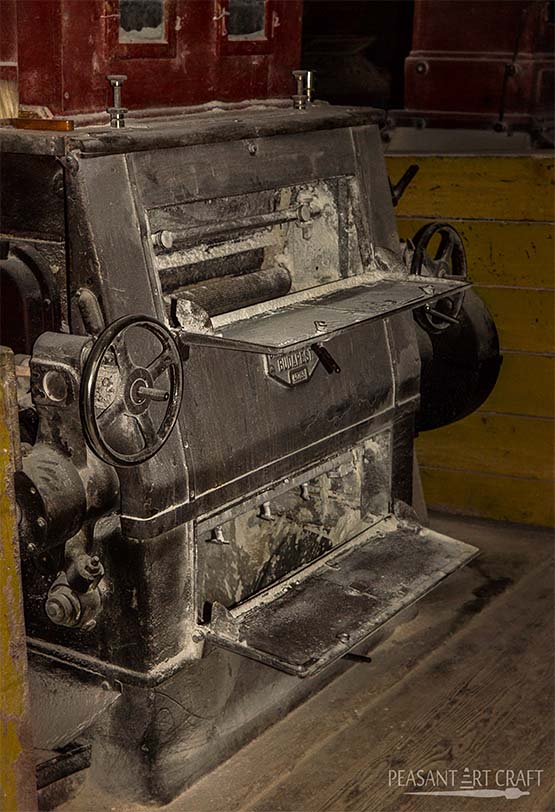The photograph captures an extremely old machine, possibly from the 19th century, situated in a dimly lit outbuilding with scratched, dusty wooden floors and brown wood plank walls that transition into a darker red painted section. The machine, standing taller than it is wide, is primarily constructed of cast iron or steel, featuring a rough, dark-colored exterior. Its structure forms a tall, four-sided shape where the front slopes back, tapering towards the top. 

The machine possesses several notable components, including a pair of wheels on either side, resembling steering wheels or valve controls. These wheels surround openings in the machine—one at the top, revealing mechanical rollers inside, and another at the bottom, with a door that swings open like an oven or furnace door, suggesting it may have been used for heating objects or materials. The interior of these compartments appears coated in ash or dust, with a whitish-gray hue hinting at prolonged disuse. Additionally, the top of the machine houses tools likely intended for securing objects in place. 

In all, the machine's intricate design, with its mechanical rollers, pistons, and potential heating elements, hints at functions that could range from industrial processes to printing press operations. The overall scene, bathed in the muted tones of metal, gray ash, and aged wood, conveys a palpable sense of historical weight and abandonment.